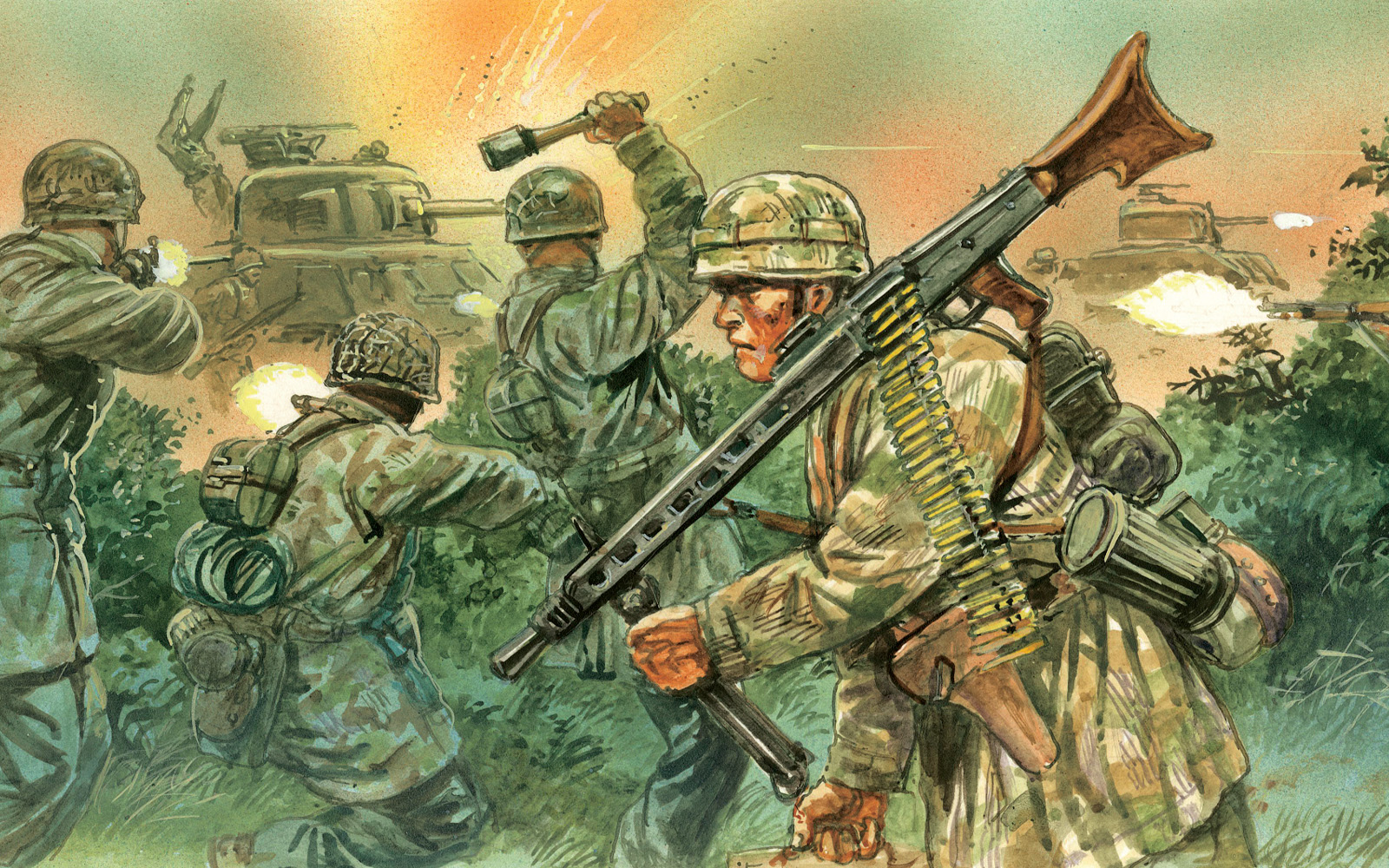This is a detailed illustration, reminiscent of a graphic novel, depicting a chaotic wartime battle. The background is predominantly green, with hues of blue interspersed, while flashes of yellow, orange, and white explode around areas of gunfire. In the foreground, a soldier clad in green and brown camouflage gear stands out. He carries a large, automatic rifle on his left shoulder, with a string of large bullets hanging from it, and is laden with additional gear. He marches from right to left, seemingly undeterred by the chaos around him. To his left, multiple soldiers, some seen from behind, engage in combat, with one holding a weapon high as though preparing to strike. In the background, tanks are visible, some firing, enveloped in the clash and firing at each other. The right side of the image also shows the fiery muzzle of another gun, adding to the scene’s intensity. Among this, one soldier hurls a grenade, contributing to the turmoil of the battle. The sky above varies between serene blue and the fiery colors of combat, enhancing the drama of the scene.